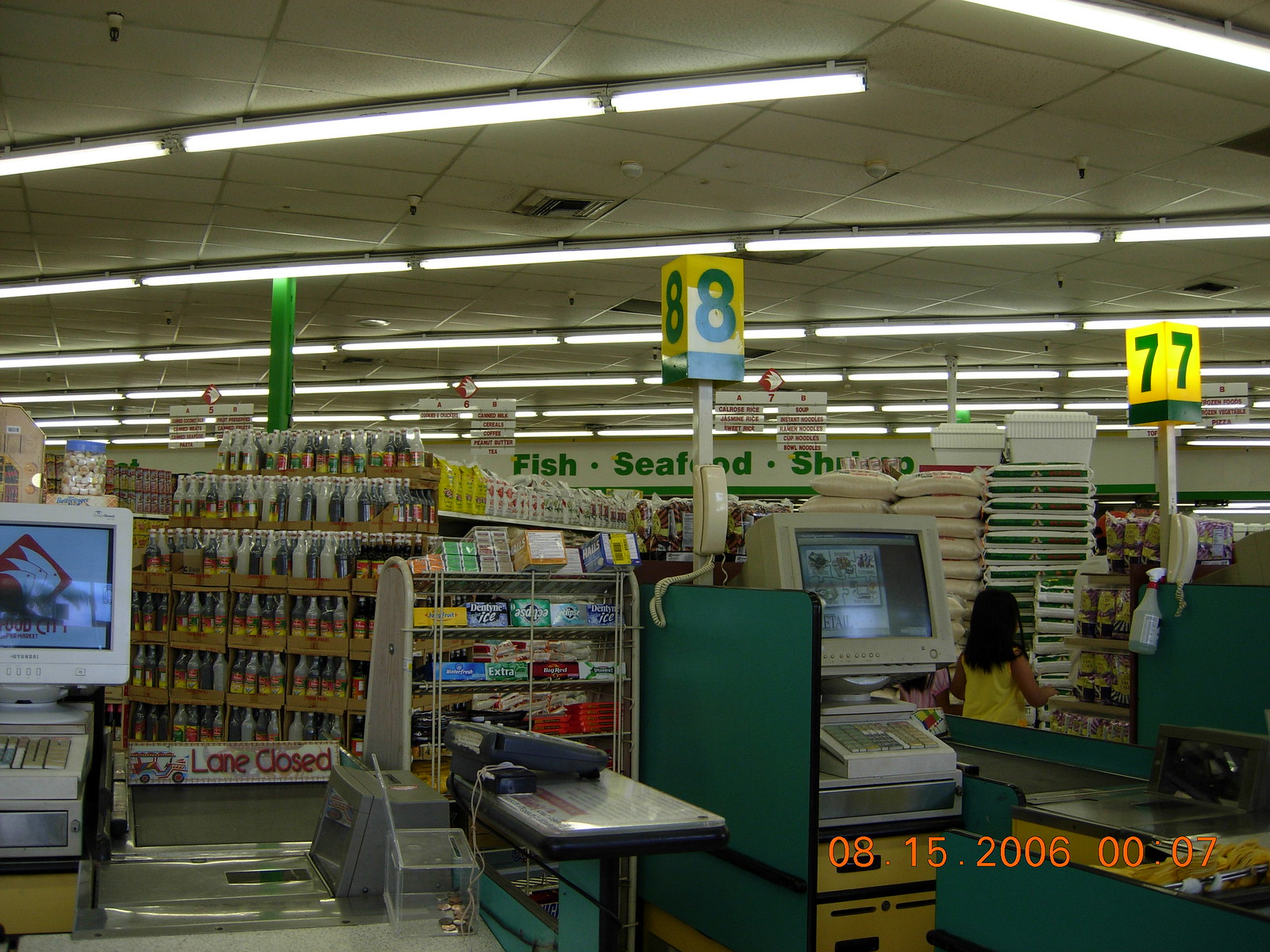This vintage photograph showcases the interior of a grocery store from behind the checkout counters, specifically tills 7 and 8. The ceiling, adorned with asbestos tiles segmented by white silver strips, is illuminated by long rows of strip lights. The checkout counters feature forest green dividers, each equipped with a computer monitor, keyboard, and money drawer. On the right side of each till, there's an elevated white platform designed for customers to place their wallets or process credit card payments.

Beyond the tills, various product display racks are visible, stocked with items like Coke, candy, and toilet paper. The back wall prominently displays the words "fish. seafood. shrimp." in green lettering against a white backdrop, indicating the seafood section of the store. The detailed layout and retro design elements evoke a sense of nostalgia, capturing a moment in time within this bustling grocery store.